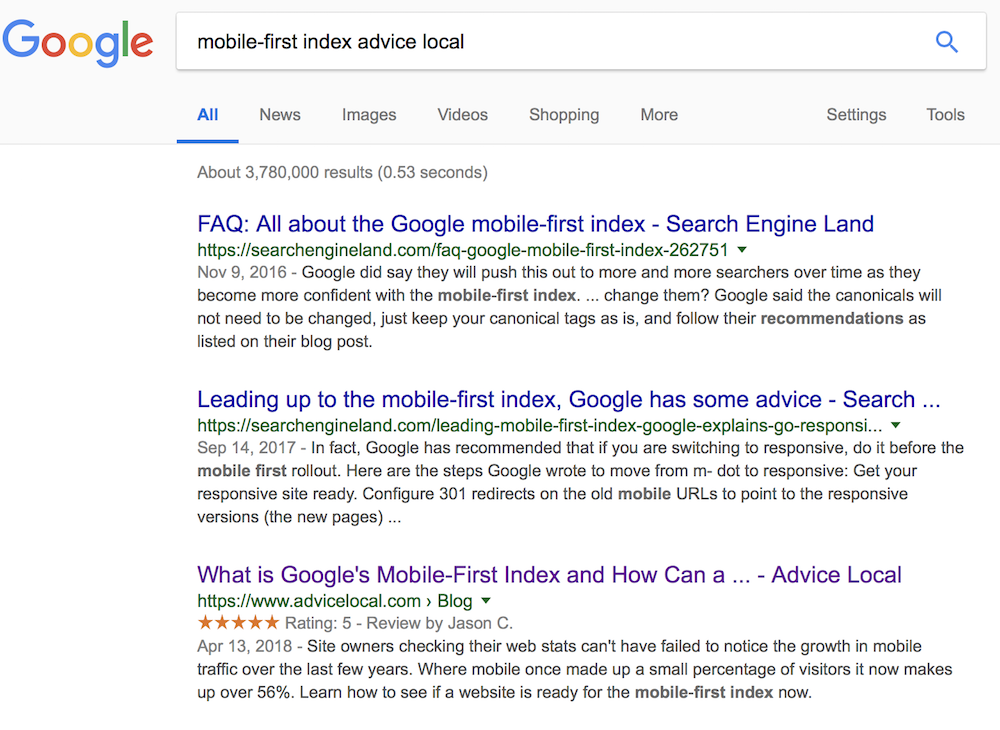This screenshot captures a Google search page featuring the query "mobile first index accuracy advice". At the top, it reads "Google", with "All", "News", "Images", "Videos", "Shopping", "More", "Settings", and "Tools" options displayed beneath. The search yields approximately 3,780,000 results in 0.53 seconds.

The first search result is a FAQ from Search Engine Land titled "All About the Google Mobile First Index" (URL: https://searchengineland.com/FAQ-Google-Mobile-First-Index), dated November 19, 2016. The snippet mentions Google's gradual rollout of the mobile first index and its advice to maintain current canonical tags without changes, following recommendations from Google’s blog post.

The second result from Search Engine Land, dated September 14, 2017, provides proactive advice for the mobile first index, emphasizing the importance of transitioning to responsive design prior to the official rollout (URL: https://searchengineland.com/leading-one-first-index-Google-explains-query-responsible). It details the steps for moving from mobile-specific URLs (m-dot) to responsive pages, including setting up 301 redirects to the new responsive URL versions.

Another highlighted result is from Advice Local's blog (URL: https://www.advicelocal.com/blog), featuring an article dated April 13, 2018, with a five-star review by JCC. It discusses the significant increase in mobile traffic, which now constitutes over 56% of web visitors, and offers guidance on preparing websites for the mobile first index.